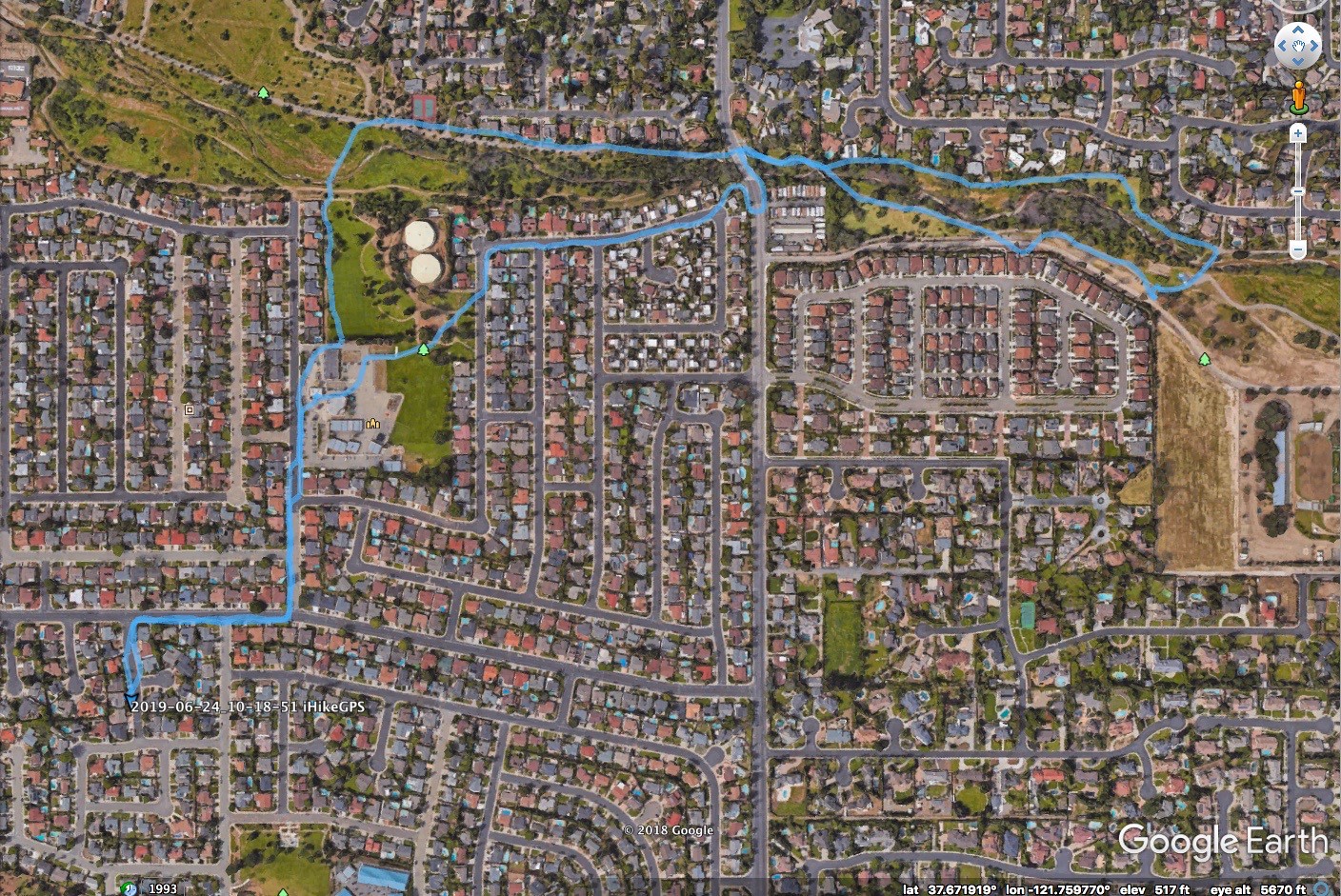In this aerial photograph, we observe a residential neighborhood captured from above. The tightly clustered houses are clearly visible, their rooftops forming a dense mosaic. Surrounding the houses, blue boundary lines demarcate different sections, accompanied by large white circular markings. The lush green grass and trees intersperse the built environment, offering a refreshing contrast to the man-made structures.

Gray roads weave through the neighborhood, connecting various parts of the area, while patches of brown earth peek through, indicating either barren lands or construction zones. In the top right corner of the image, a directional circle with arrows pointing in all four cardinal directions (up, left, right, and down) is visible, likely serving as a navigational aid.

A small yellow object can be seen within the scene, though its specific identity remains unclear. Below the main image, the text "Google Earth" is prominently displayed along with a series of numbers: 37871819 and ION 121. The clarity and vibrant detail of this Google Earth image provide a comprehensive overview of the neighborhood’s layout and features.